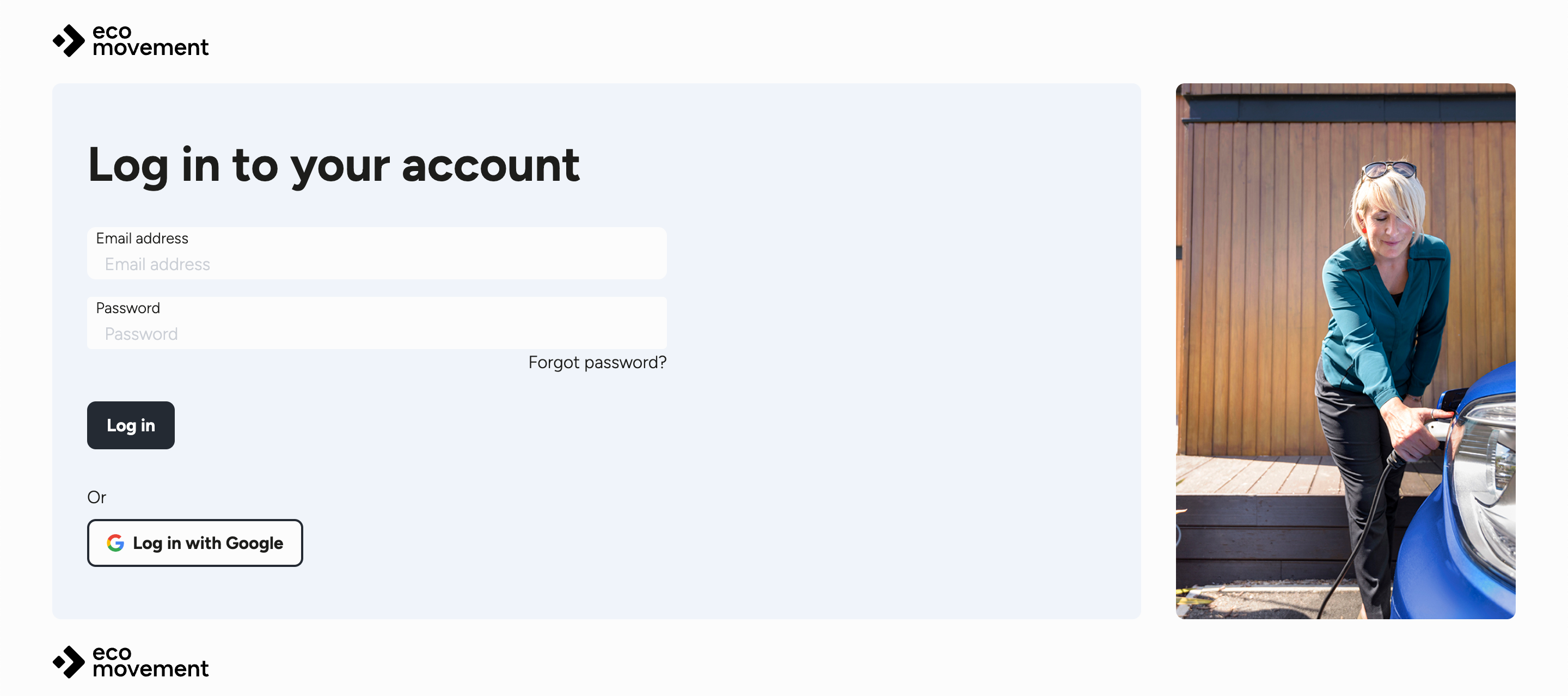**Image Description: Login Screen for 'Eco Movement' Website**

The image displays a login screen for the "Eco Movement" website. The background is primarily light gray. 

1. **Top-left Corner:** 
   - A small symbol is present.
   - "eco movement" is written in black, lowercase letters next to the symbol.

2. **Central Section:**
   - A darker gray box with the title "Log into your account."
   - Below this, there are two text fields:
     - The first field is for entering an email address.
     - The second field, located beneath the email field, is for entering a password.
   - At the bottom right corner of the password field, there is a text link that says "Forgot password?"  This is likely for users who need to reset their password.

3. **Bottom Section of the Login Box:**
   - There is an option to log in.
   - Additionally, there is an option to log in with Google.

4. **Right Side of the Login Information:**
   - A picture of a woman fueling a car:
     - The car appears blue, and only the top, first headlight, and fuel hose are visible.
     - The woman is placing the fuel hose, which might be an electric charging cable given the "eco" context, into the car.
   - The woman has short blonde hair with sunglasses resting on top of her head.
   - She is wearing red earrings, black pants, and a long-sleeved, blue-green sweater.